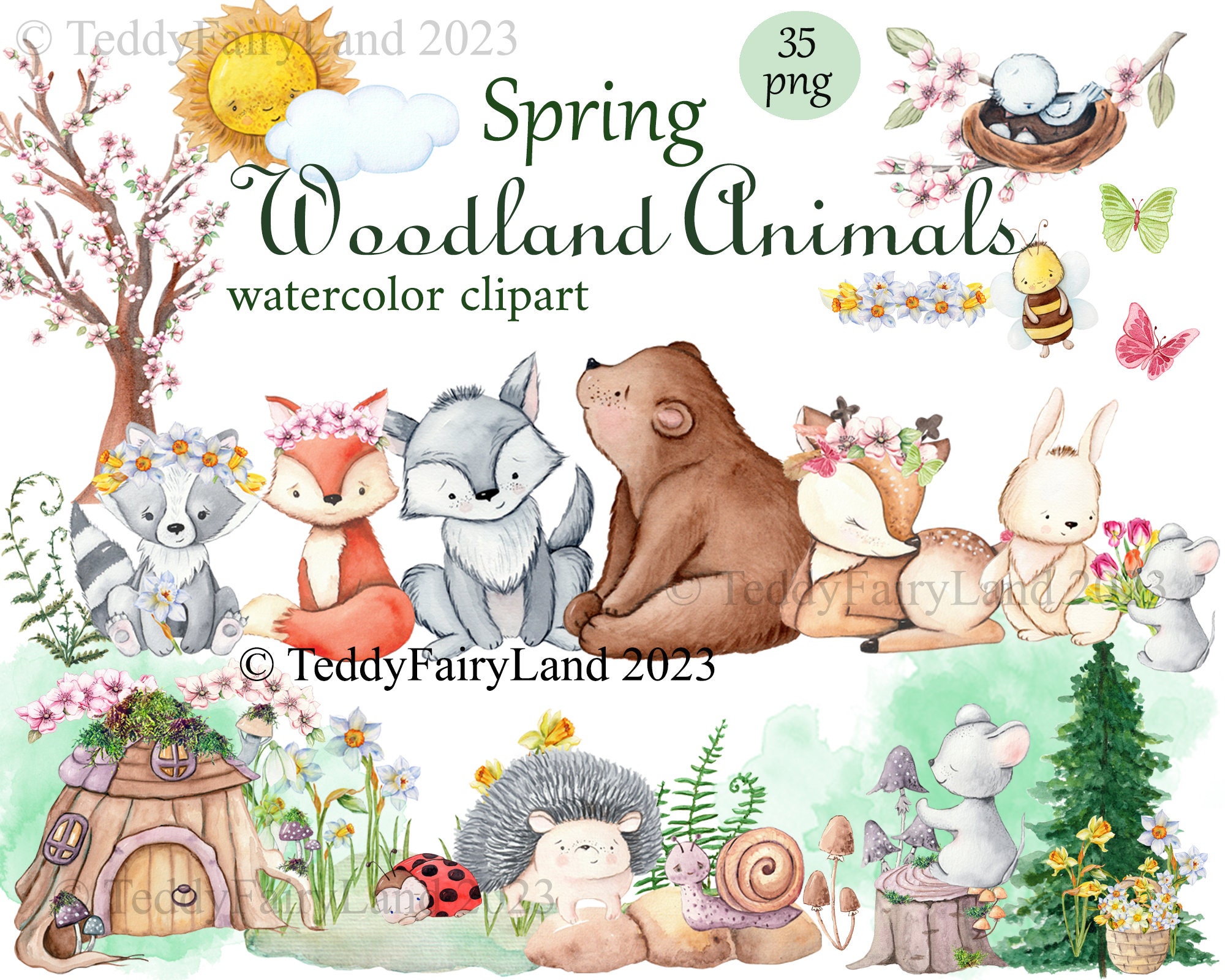This image is a detailed watercolor clip art titled "Spring Woodland Animals," copyrighted by Teddy Fairyland in 2023. The illustration contains 35 digital PNG characters with soft, welcoming colors, suitable particularly for children. Amongst the many woodland creatures are bears, foxes, deers, raccoons, rabbits, and a mouse, as well as a variety of insects like bees, butterflies, ladybugs, and snails. The scene is set in a whimsical, fictional forest featuring a tree house, flowers, ferns, and a smiling sun peeking from behind a cloud. Animals are adorned with crowns of cherry blossoms and narcissus daffodils; the raccoon holds a bluish flower while the fox, wolf, and bear sit thoughtfully. A bunny accepts a bunch of flowers from a mouse, and a cottage made from a tree stump with mushrooms and flowers add to the enchanting setting. Additionally, there are humanized creatures like a bee with a little face, ladybugs, and a snail. The overall illustration exudes a charming, fairy-tale atmosphere with vibrant, delicate details.